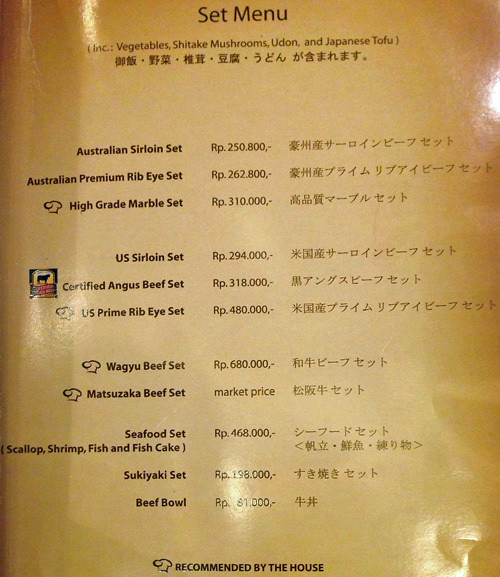The image depicts a glossy yellow restaurant menu with a soft beige and tan sheen, primarily featuring a "Set Menu" at the top. This section includes vegetables, shiitake mushrooms, udon, and Japanese tofu. The menu text is written in both English and Japanese. Below the initial descriptions, a variety of dish options are listed with their prices. These include the Australian Sirloin Set (RP 250,800), Australian Premium Ribeye Set (RP 262,800), High Grade Marble Set (RP 310,000), U.S. Sirloin Set (RP 294,000), Certified Angus Beef Set (RP 318,000), U.S. Prime Ribeye Set (RP 480,000), Wagyu Beef Set (RP 680,000), Matsuzaka Beef Set (market price), Seafood Set offering scallops, shrimp, fish, and fish cake (RP 468,000), Sukiyaki Set (RP 198,000), and Beef Bowl (RP 81,000). At the bottom of the menu, there's a symbol indicating "Recommended by the House." The menu's text is predominantly black against the tan background, and the overall layout is centrally positioned within the photograph, emphasizing the list of food items and prices.